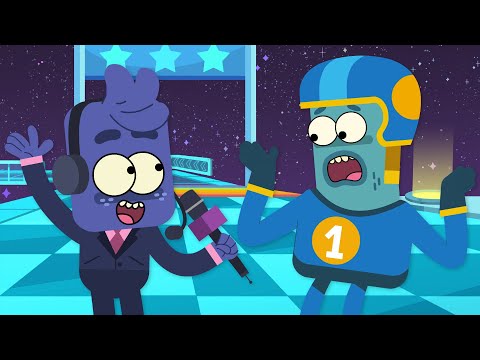The image is a rectangular frame from a cartoon, complete with letterbox-style black spaces at the top and bottom. The scene is set against a dark, purplish-black space sky dotted with white stars. Dominating the center is a racetrack field featuring a checkered pattern in alternating dark blue and light blue squares. A finish line, marked by two poles, holds up a blue sign adorned with white stars.

On the left side of the racetrack, a sportscaster character with a rectangular, purple head and bulging white eyes is shown holding a microphone and wearing a headset. He appears to be interviewing another character who is wearing a blue football helmet with a light blue stripe and an orange oval. This helmeted character also has large white eyes, and he dons a blue jersey featuring a number one inside an orange circle. The athlete's mouth is open, and his body language, with hands raised, suggests he is either surprised or perplexed.